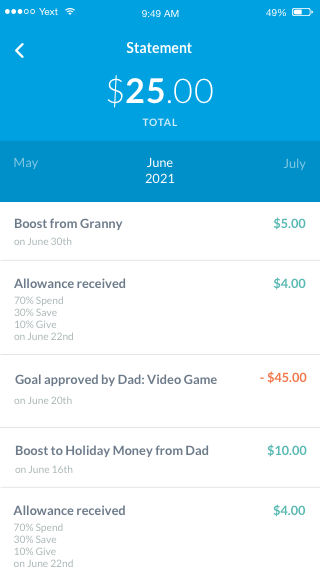A detailed snapshot of a finance tracking app displayed on a mobile phone in portrait orientation:

The image captures the interface of a financial app with a clean user interface divided into distinct sections. The top third of the image is dominated by a blue header. Within this header:

- Five small dots are positioned in the top-left corner, with three out of five dots highlighted, possibly indicating the user's progress.
- The app name "Yext" is displayed next to these dots.
- Following this, various status icons are shown: a Wi-Fi signal indicator, the current time "9:49", and a battery status showing 49% charge remaining.

Beneath this header lies another blue section where the app prominently displays a "Statement" with a total amount of "$25."

Immediately below, in a slightly darker blue, is a navigation bar with the months "May," "June," and "July." "June" is highlighted, indicating the current selection.

The main body of the image, which is white, lists various financial transactions in chronological order. It includes:

- "Boost from Granny on June 30th" marked as $5 in green.
- "Allowance received" of $4 in green with an allocation breakdown of "70% spend, 30% save, 10% give" on June 22nd.
- "Goal approved by Dad, video game" noted as a deduction of $45 on June 20th.
- "Boost to holiday money from Dad" contributing an additional $10 on June 16th.
- Another entry for "Allowance received" displaying similar allocation percentages and an amount of $4.

This detailed snapshot effectively communicates the app's user-friendly interface, highlighting various inputs such as allowances, financial goals, boosts from family members, and their respective distributions.